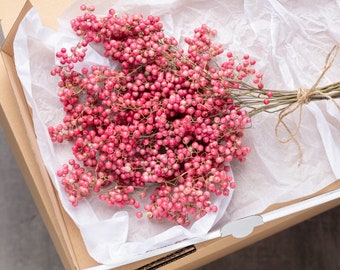The image is a detailed color photograph of a sizable cluster of reddish-pink berries attached to green stems, resembling an abundant bouquet. Each branch is densely packed with hundreds of round berries, creating the appearance of a vibrant, botanical arrangement. The stems are tied together neatly with twine, giving the whole bundle a natural, rustic look. This entire arrangement is set inside a shallow wooden box or tray, which is lined with white tissue paper. The box itself rests on a surface that is partially visible, showing small grey triangles in the lower left and right corners of the photograph. The precise details and overlapping descriptions emphasize the vivid colors and the thoughtful presentation of the berries within the box.